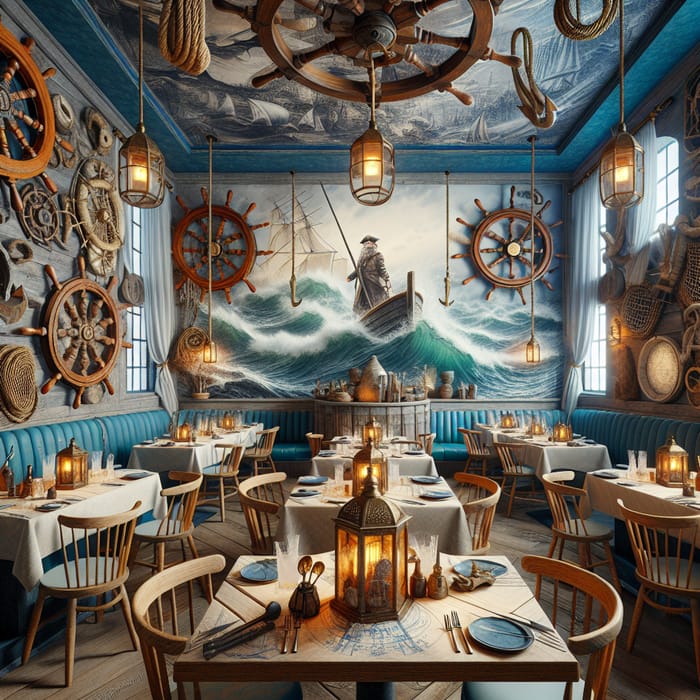This illustration portrays the interior of a nautical-themed restaurant. The dining area features a mix of tables arranged in three rows, including individual tables and one long communal table, each adorned with metal lantern centerpieces and blue plates alongside neatly placed silverware. The seating comprises wooden chairs with curved backs and blue booth seats lined along the walls. Decorative ship's wheels of varying sizes and colors hang on the left wall, while the back wall showcases a mural depicting a man in a small boat with a larger ship in the background, reminiscent of a Captain Ahab scenario. The right wall is festooned with fishing nets and other maritime paraphernalia. Overhead, a ship's steering wheel chandelier complements the nautical motif, with ropes hanging down to support lights. Natural daylight filters into the dimly lit room, highlighting the restaurant's wooden flooring and creating an ambiance that vividly mirrors an old, seafaring vessel.